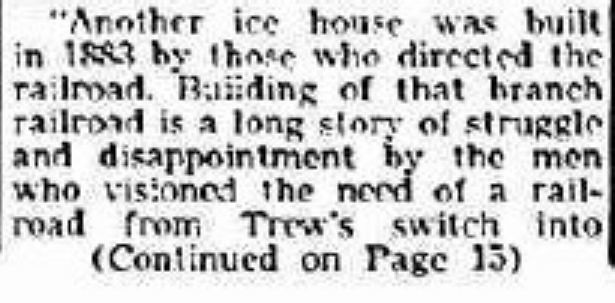The image shows a somewhat blurry text excerpt from a newspaper article, bordered by vertical and thicker black lines, with portions of the text appearing faded as if from a malfunctioning typewriter. The text recounts a piece of historical information: "Another ice house was built in 1883 by those who directed the railroad. Building of that branch railroad is a long story of struggle and disappointment by the men who visioned the need of a railroad from True Switch into..." followed by "(continued on page 15)." The article describes the challenges faced by the men who oversaw the construction of a spur railroad line, crucial to connecting an outlying area to the main rail network.